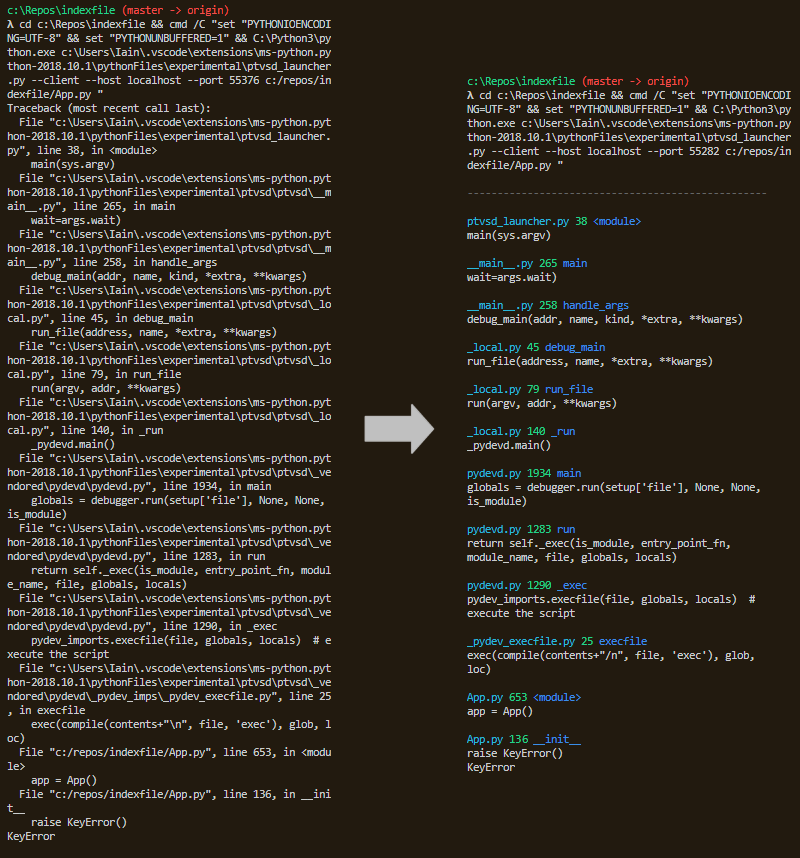An initial glance at the image reveals a stark contrast between chaotic and organized code. On the left side, there's a mass of poorly spaced text in predominantly white color, displaying complex file paths such as `C:\Users\InVain\VSCode\extensions\mspython\PTY-HH-18.10.1`, clearly indicating it's Python-related. Additionally, specific file markers like `C repros index file`, `master`, `forward origin` in red, and `repros index file` in green, accompanied by a right-pointing arrow, signify code changes and version control states.

On the right side of the image, we see a neatly recompiled version of the jumbled code. This reformatted code includes clear syntax with components like `PTVSED_Launcher`, `System_RG`, `local_PV1-40`, and an error-handling line `raise KeyError` towards the bottom. The refined Python code is significantly more readable and appears to function without the clutter observed on the left. 

Above the restructured code snippet on the right side is a section of the original code retained as a reference point, emphasizing the transformation undertaken. The overall impression of the image is that someone has diligently reorganized and simplified a chaotic chunk of code into an efficient, functional Python script.